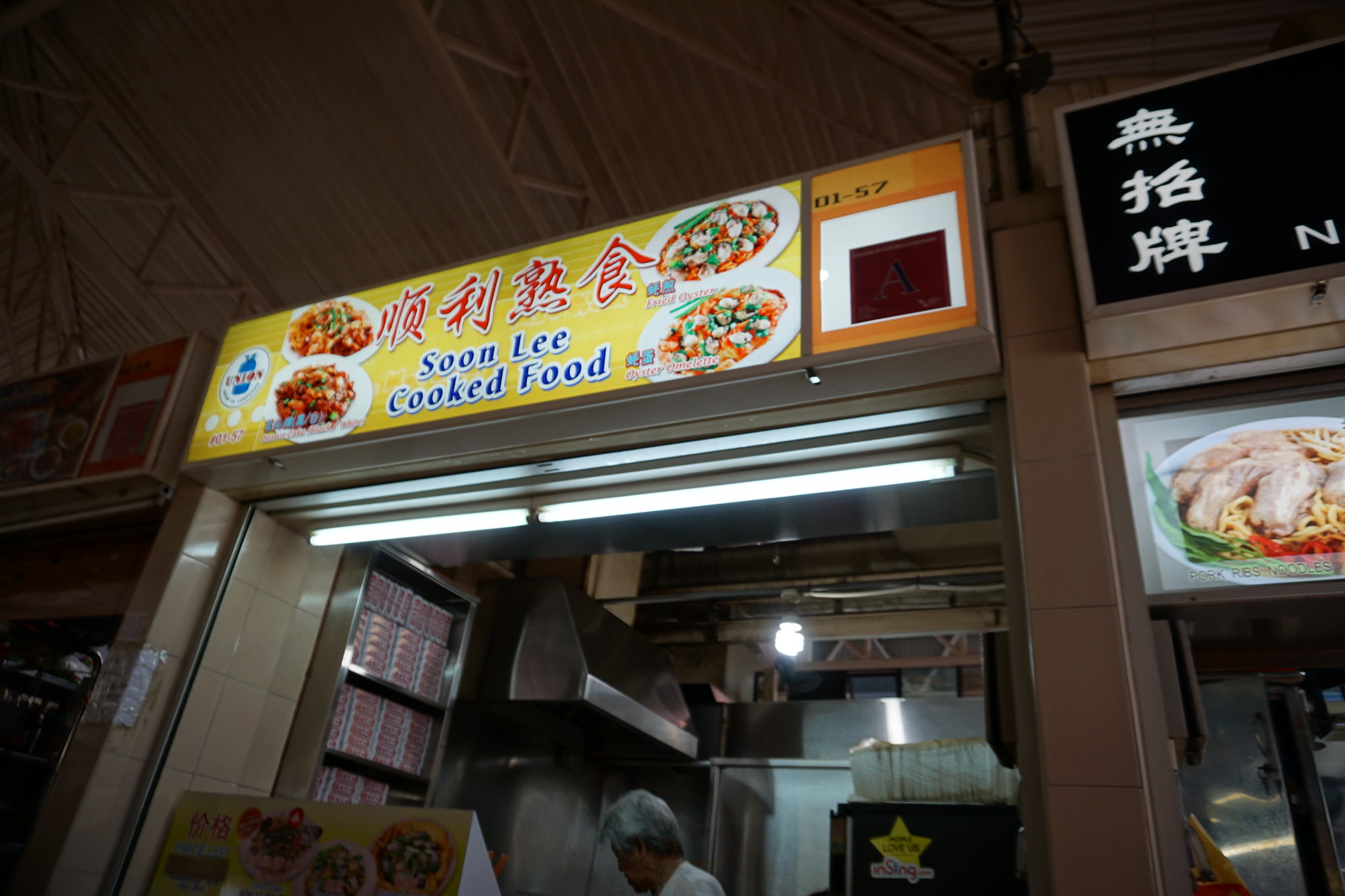The photograph depicts an oriental food stall, prominently centered in the image, with the name "Soon Lee Cooked Food" displayed in blue text with a white outline and black shadow on a large, illuminated yellow sign. Above the name, red text in Asian characters indicates the likely setting to be somewhere like South Korea or Japan. The stall is part of a row of similar stalls, suggesting a busy food court or street food market. To the left and right, there appear to be other food offerings, including dishes that look like chicken and shrimp or oyster soup.

Inside the stall, an older Asian man with gray hair can be seen cooking on a silver stovetop, with a large silver oven hood above him. The confined cooking area includes a counter indicating it's more likely a fast food takeaway than a sit-down restaurant. Visible on the left side inside the stall is a pile of boxes, presumably used for food packaging. The space is lit with strip lighting, indicating an indoor environment like a shopping mall or a dedicated food market area. The photograph appears to be taken on a smartphone, reflecting an amateur but good-quality shot.